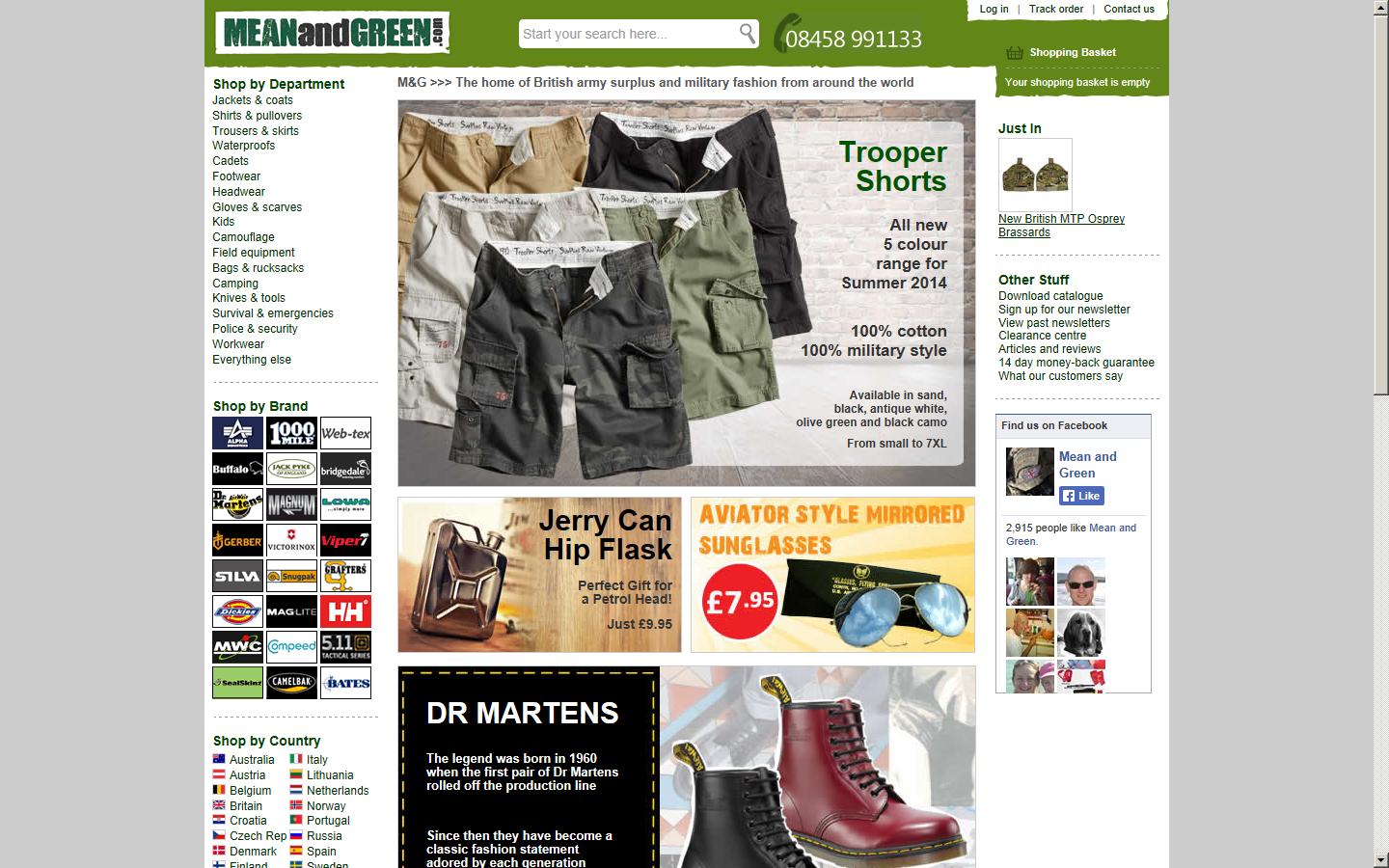In the image, the top left corner features a logo for "meanandgreen.com," where "mean" and "green" are in green text, while the rest of the text is in black, all set against a white rectangle. Adjacent to this on the right is a search bar with the placeholder text "Start your search here" and a magnifying glass icon on the far right. 

In the top right corner, the navigation menu includes three categories: "Contact Us" on the far right, "Your Order" to its left, and "Log In" further to the left.

Dominating the center of the page is a large square image showcasing several pairs of shorts in a variety of colors, including black, white, brown, green, and dark black. To the right of this main image, the product is named "Trooper Shorts," with text below advertising the shorts as an all-new five-color range for summer 2014, made from 100% cotton and styled in a military fashion.

Below this central section, there are smaller boxes featuring advertisements for other products. Highlighted among these is the "Jerry Can Hip Flask" and "Aviator Style Mirrored Sunglasses," with the latter priced at $7.95.